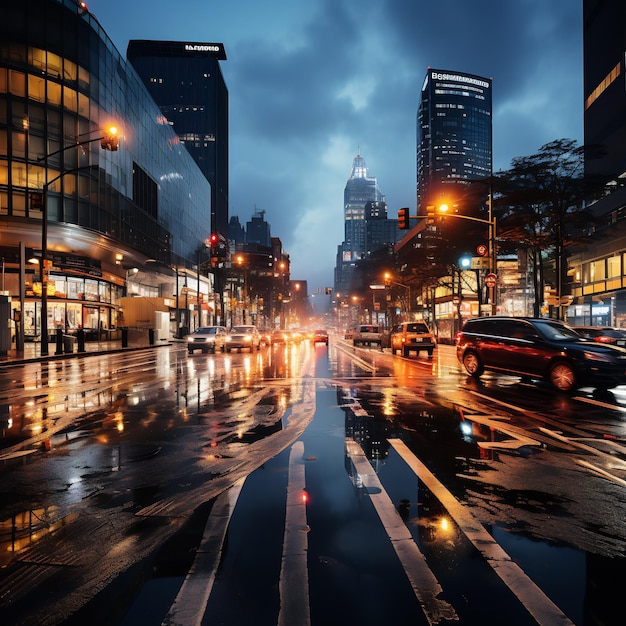This photograph captures a city street at night after a recent rain, with a perspective from the middle of the street among gleaming wet surfaces. The wet pavement reflects the bright lights of street lamps and vehicles, giving the street an almost glowing appearance. The intersection ahead features a crosswalk, and the headlights of stationary cars at a red light dominate the scene, creating a striking effect. On either side of the street, tall buildings, possibly businesses, are brightly lit, with some floors illuminated and others dark, showcasing the varied occupancy. Notable is a glass building on the left and additional towering skyscrapers framing the image on both sides, their tops shrouded in darkness with intermittent lights. Trees can be seen lining the street, adding to the urban landscape. The sky above is filled with overcast, dark gray clouds, contributing to the dramatic ambiance. In the distant background, another skyscraper appears partially cloaked in fog, enhancing the city's nightscape.